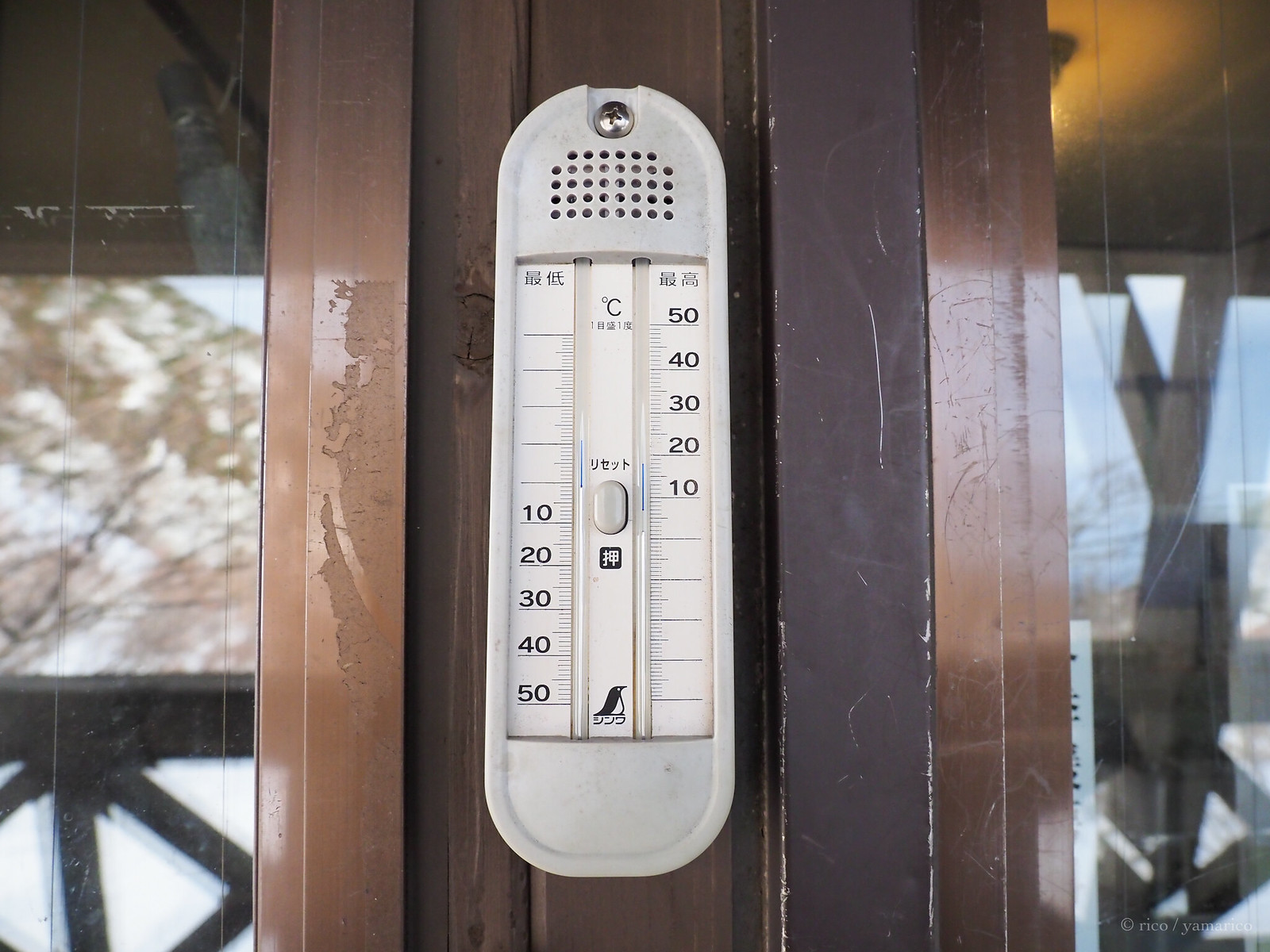This outdoor photograph captures a serene winter scene on a patio deck. Flanked by two windows on either side, their reflective surfaces reveal the snowy trees and the brown deck railing adorned with crossbars. The focus of the image, however, is a prominently displayed white metal thermometer with distinctive Asian characters at the top left, middle, and top right sections.

Embedded at the center of the thermometer, just above the Asian characters, is a small "C" within a circle, signifying Celsius readings. The thermometer also features a white, pill-shaped button whose function remains unclear. Numerals are clearly marked along both sides of the thermometer: the left side ascends from 10 to 50, while the right side descends from 50 to 10. The brown wooden frame of the patio and the thermometer's placement against this frame contribute to the rustic, yet precise, ambiance of this wintry outdoor setting.